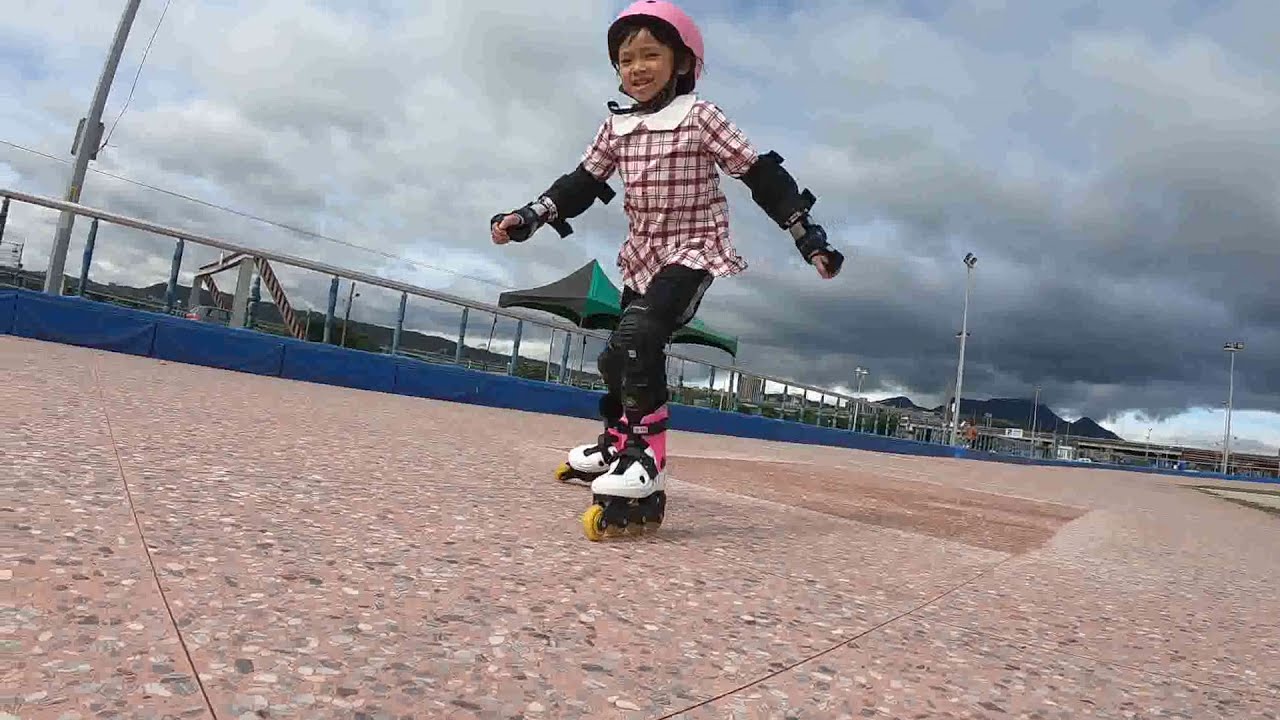This image showcases a young girl, possibly of Asian descent, roller skating on a park or boardwalk with a granite floor composed of various tiny stones. She sports a pink helmet with a black chin strap and has black hair with bangs peeking out. The girl is dressed in black pants with black knee pads and a white-and-purple blouse featuring a white collar. Both of her arms are protected by black elbow and wrist pads. Her roller skates are vibrant pink and white with yellow reels. Surrounding her is a railing lined with blue pads, and in the background, the sky is a light blue adorned with a few clouds. The granite pathway she skates on has a pale pink, beige, and gray hue. The scene is accented by the fence and poles that can be seen in the backdrop, adding a few subtle pops of color to this otherwise neutral setting.